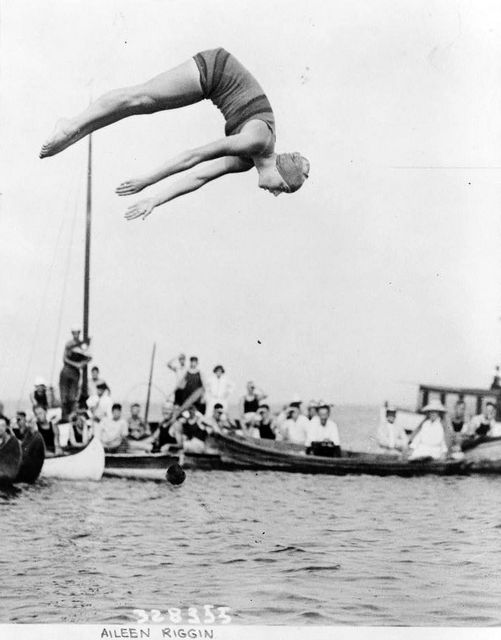This vintage black and white photograph captures an iconic moment in diving, featuring a woman identified as Aileen Riggin in mid-dive. Aileen, a white woman, is gracefully captured in a pike position—her legs are extended straight out, toes pointed, arms stretched in front of her, with her head rolled back, gazing down towards the water she is about to enter. The scene unfolds against the backdrop of a body of water, possibly a river or ocean, where numerous boats and canoes, populated with around 20 spectators, keenly watch her impressive dive. Among these boats, one sailboat stands out, with a man holding onto a pole, adding depth to the scene. The photograph is annotated at the bottom with her name, "Aileen Riggin," and the code "328355," lending a documentary feel to the composition.